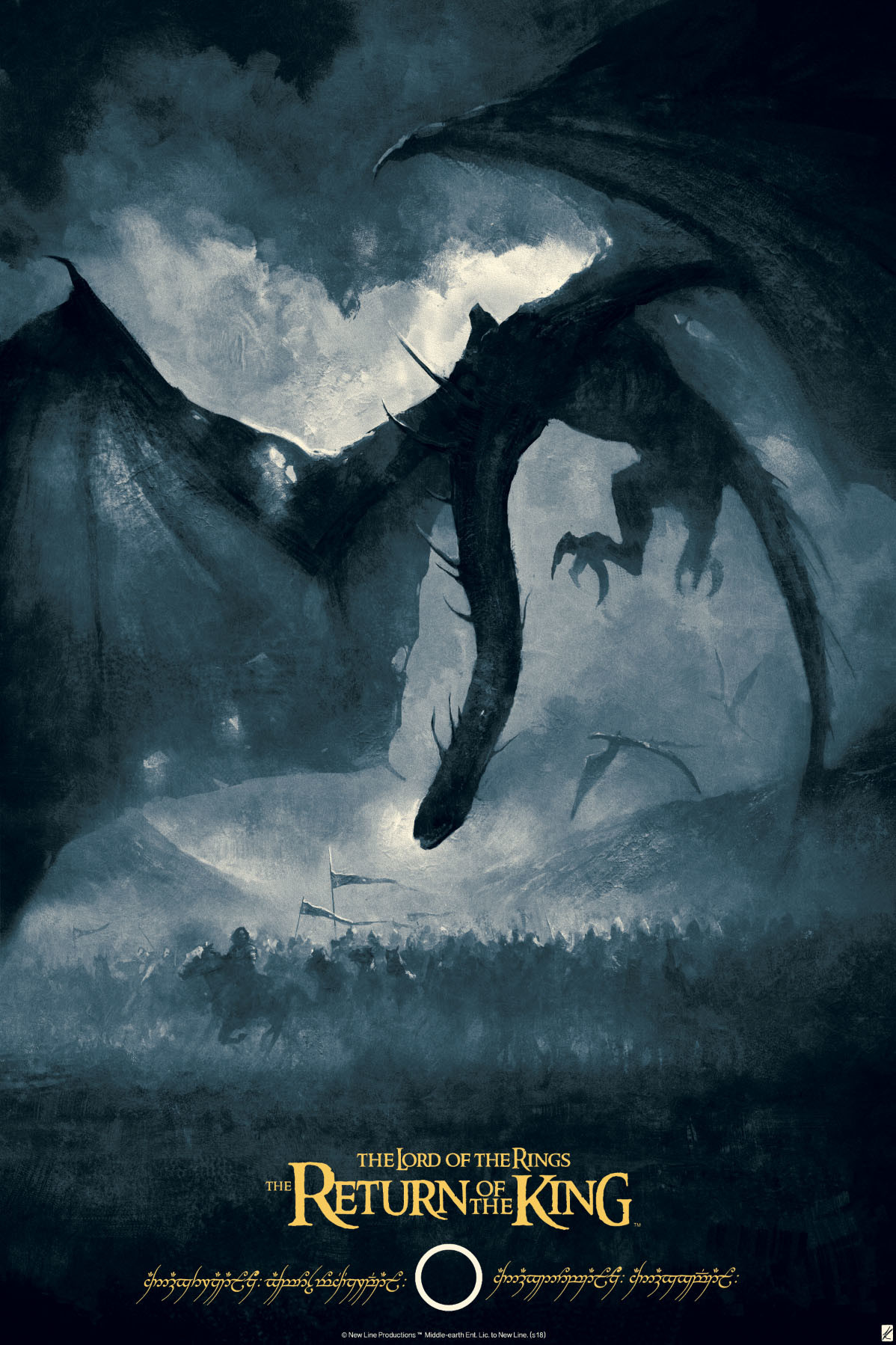This poster for "The Lord of the Rings: The Return of the King" features a monochromatic palette dominated by various shades of grey, accented with touches of white. At the center of the image is a colossal, dragon-like creature in mid-flight, its expansive wings stretching from one side of the poster to the other. The beast's elongated tail trails behind it, while its partially extended legs and outstretched claws suggest it is poised to descend upon the figures below. In the backdrop, more similar creatures can be seen soaring through the sky.

Below the monstrous figure, a large group of men on horseback charge across an open field, their gallant steeds adorned with fluttering flags. The atmosphere above is laden with greyish clouds, tinged with slight hints of white, contributing to the overall sombre and foreboding mood of the scene.

The title "The Lord of the Rings: The Return of the King" is prominently displayed in bold yellow letters at the top of the poster. Below the title, there is a line of text in a script that could be mistaken for Arabic or an Indian script, though its precise nature is indistinct. A small copyright notice appears at the very bottom of the poster, although its minuscule size makes it difficult to decipher.